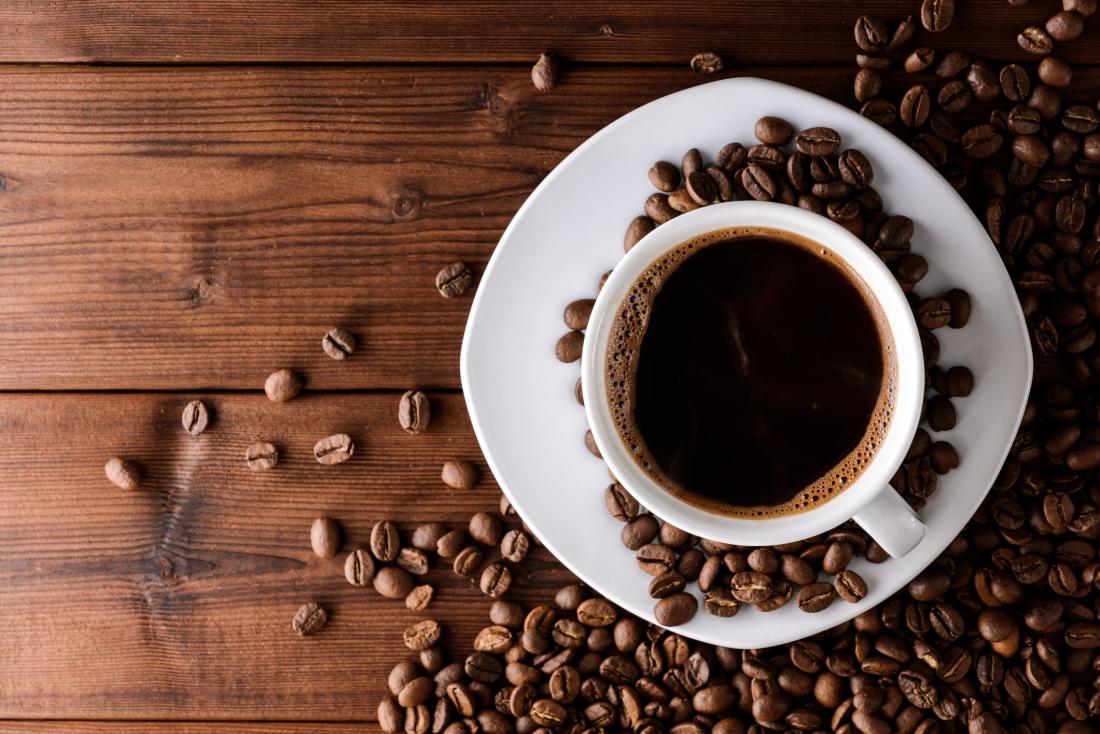This top-down image captures a rich and aromatic coffee scene from an overhead angle. At the center, a dark coffee fills a white mug, showing a few delicate bubbles on its surface, indicating it is freshly brewed. The cup rests on a matching white plate that lies on a brown wooden table with visible grain patterns and a polished finish. Surrounding the cup and plate is an abundance of coffee beans, predominantly concentrated on the bottom right half of the image. These beans, some whole and some split, scatter densely under and around the plate, extending towards the left side but becoming less frequent as they spread, leaving the top left corner of the image mostly clear, revealing the natural texture of the wooden table.